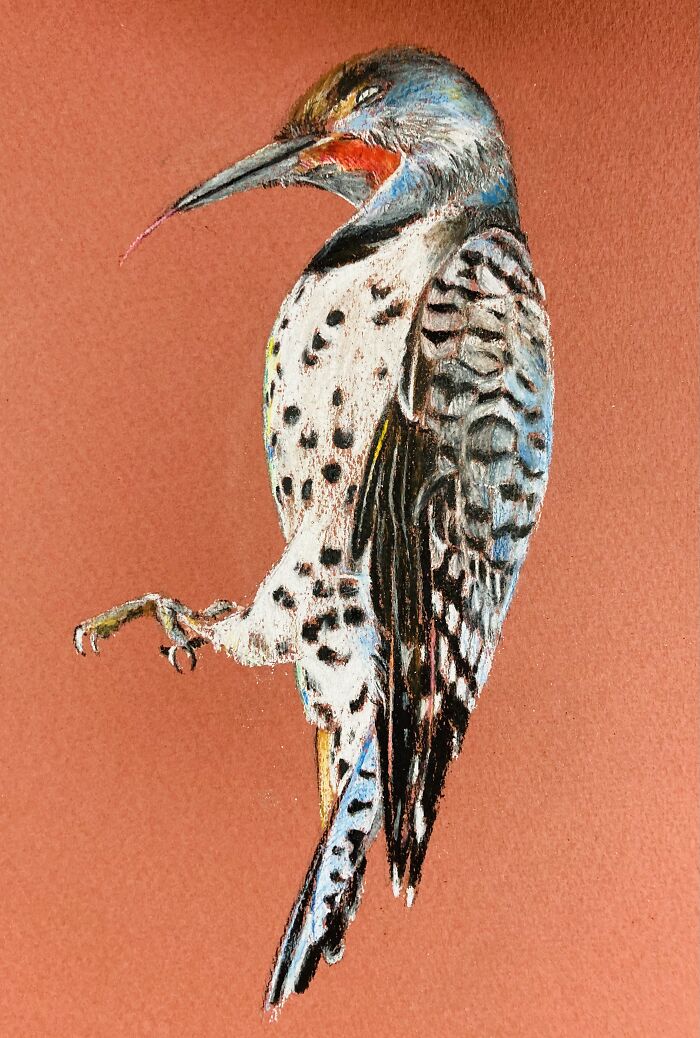This captivating vertical illustration showcases a woodpecker poised against a muted terracotta orange canvas. The bird, rendered either in acrylic or oils, dominates the center of the image. Its vibrant head features a striking combination of colors: a blue hue on the lower part and yellow on the top, with a red streak running from its neck to its slender, gray beak. The beak, pointed and elongated, holds a delicate, pink worm. The bird's small white eye adds a touch of sharpness to its keen expression.

The woodpecker's body is primarily white, adorned with black specks along its chest. Its wings are a blend of blue, gray, and cream tones, with black-tipped feathers that reveal a meticulous attention to detail. The claws, appearing to grasp an invisible perch, are splayed out towards the left side of the canvas, almost two-thirds down from the top. The tail feathers extend gracefully towards the bottom edge of the image.

Overall, the painting captures the essence and beauty of the woodpecker with its intricate details and rich palette, set against a warm, earthy backdrop, highlighting both the delicate and the striking features of this fascinating bird.